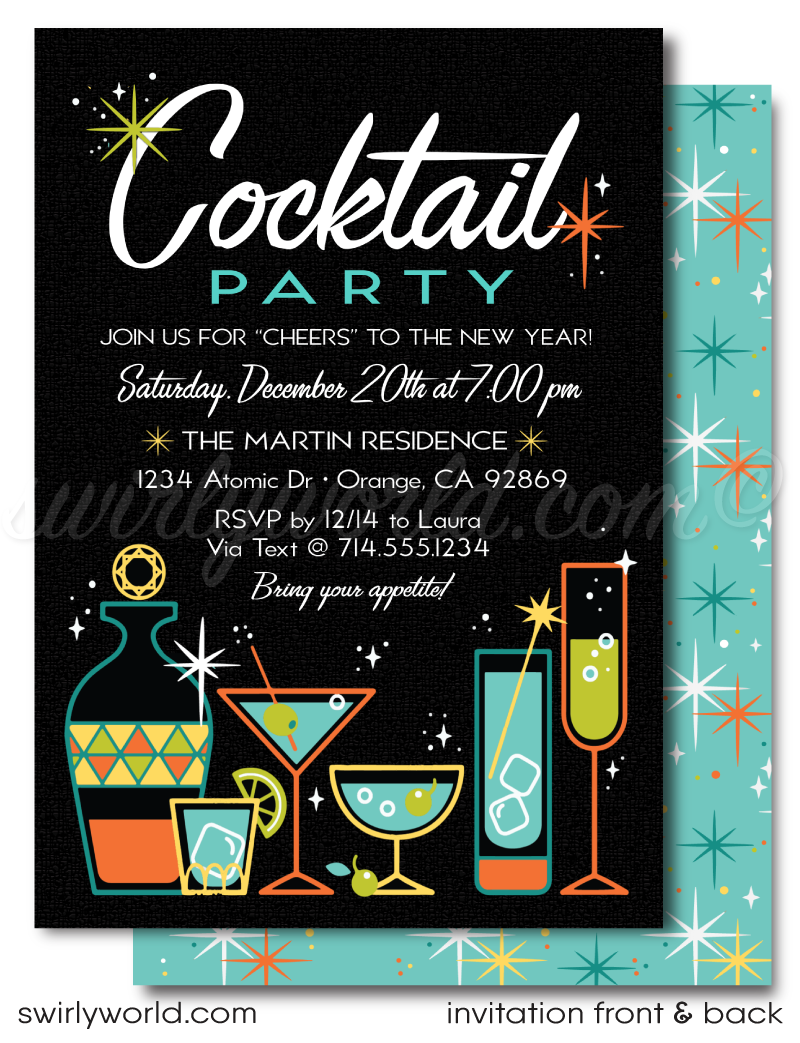The image displays a colorful and festive invitation for a cocktail party, with both the front and back of the invitation visible. The back side is a light green background adorned with vibrant blue, white, orange, and yellow starbursts that criss-cross dramatically. Some of these starbursts feature long vertical lines through their centers. Additional design details show the text "swirlyworld.com." 

The front of the invitation, which is overlaying part of the back, has a striking black background that showcases white and blue text. The heading "cocktail party" stands out in large, bold letters— "cocktail" in white and "party" in blue. Below this, the invitation reads: "Join us for cheers to the new year, Saturday, December 20th at 7 p.m. The Martini Residence, 1234 Atomic Drive, Orange, CA 92869. RSVP by 12-14 to Laura via text at 714.555.1234. Bring your appetite!" 

Additionally, images of champagne glasses, martini glasses, and other bottles are artfully arranged at the bottom, enhancing the celebratory theme of the invitation.